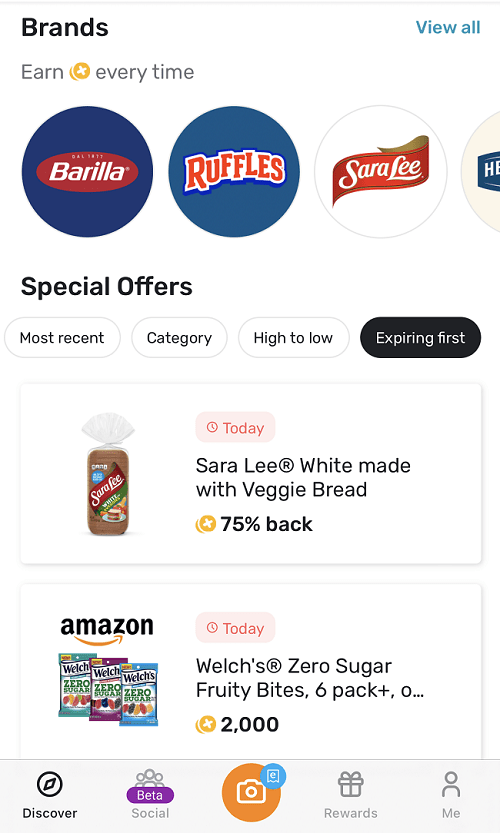This detailed screenshot captures the interface of a food ordering page dedicated to grocery shopping, highlighting various elements and offers available to users.

In the top left corner, the page prominently displays the section title "Brands." Just beneath this, there's a small text that reads "Earn every time" accompanied by an icon of a gold coin, indicating a rewards program.

The page features three logos displayed in a row, representing different brands: Barilla, known for its spaghetti products; Ruffles, the popular snack brand; and Sara Lee, renowned for its bakery items.

Beneath these logos, the page includes a section titled "Special Offers." Under this heading, there are four categorization tags that help users sort through the offers: "Most Recent," "Category," "High to Low," and "Expiring First," with the "Expiring First" tag highlighted in a black bubble.

The next part of the page is divided into two product sections. The first showcases "Sara Lee White Made with Veggie Bread" with an enticing offer of "75% back" and a tag marked "Today" indicating immediate availability. The second product listed is "Welch's Zero Sugar Fruity Bites Six Pack" from Amazon, valued at 2,000 coins, and also features a red "Today" tag.

At the bottom of the page, a navigation bar contains five icons. The first icon, labeled "Discover," is represented by a circle with a slanted diamond inside. The second icon, "Social," depicted by a paw print with a purple oval marked "beta." Next, there's an orange camera icon. Following that, the "Rewards" section is symbolized by a gift box. Lastly, the profile section is denoted by the silhouette of a person.

The comprehensive layout and various elements suggest an intuitive and rewarding shopping experience for users looking for their favorite grocery items while also taking advantage of special offers and rewards.